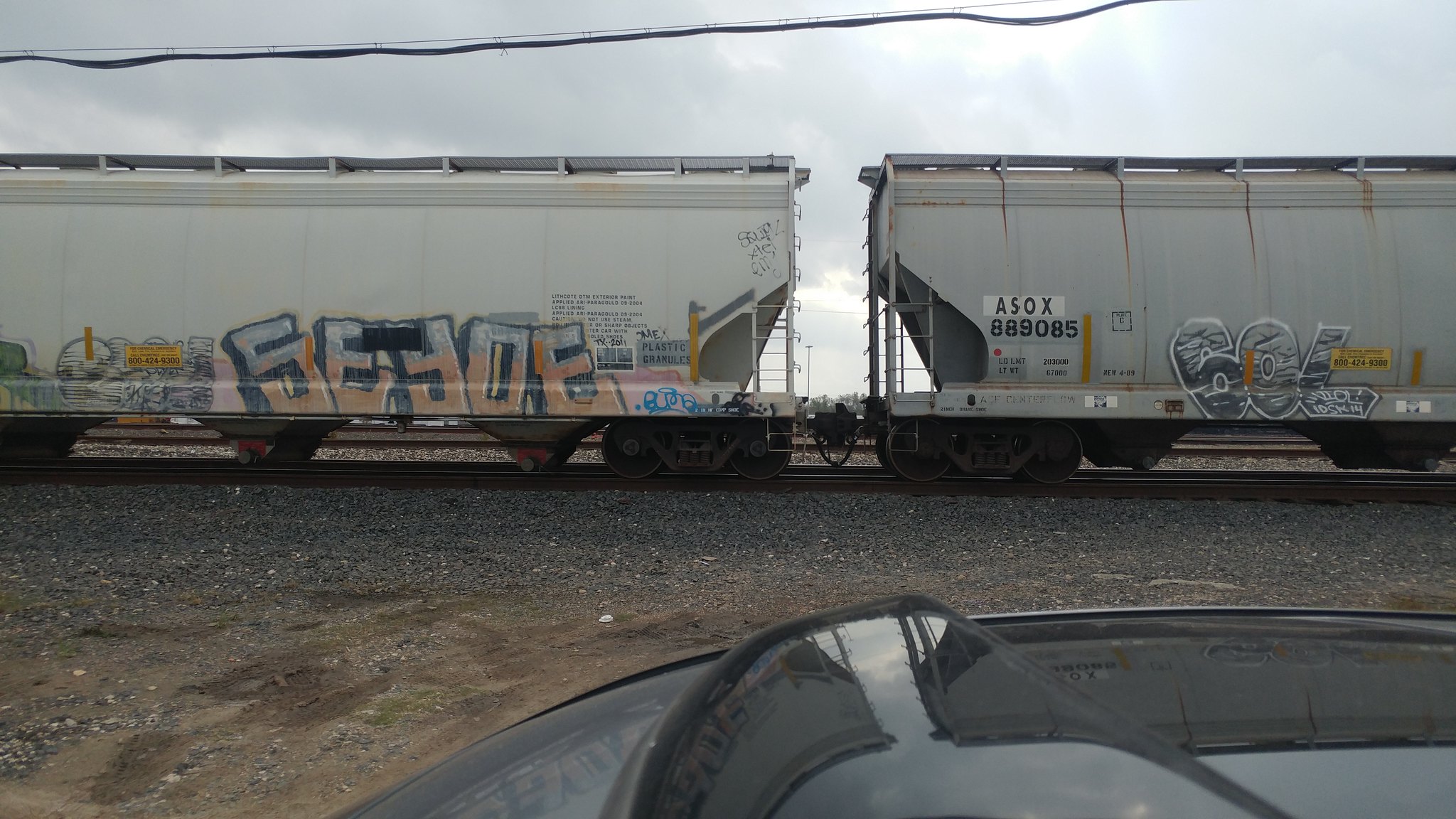This photo, taken from inside a black car stopped at a railroad crossing, showcases two long, white train cars covered in vibrant graffiti with large block letters in blue, orange, and black scrolls. The enclosed train cars, likely used for transporting grains, sit on tracks that are set into a gravel and dirt foreground, peppered with small pebbles. The scene is framed by a partially cloudy blue-gray sky with sunlight breaking through, highlighting a black telephone wire stretching across the top of the image. Visible in the foreground is a patch of damp, brown dirt beside the car's hood and sunroof, adding depth and realism to the photo.